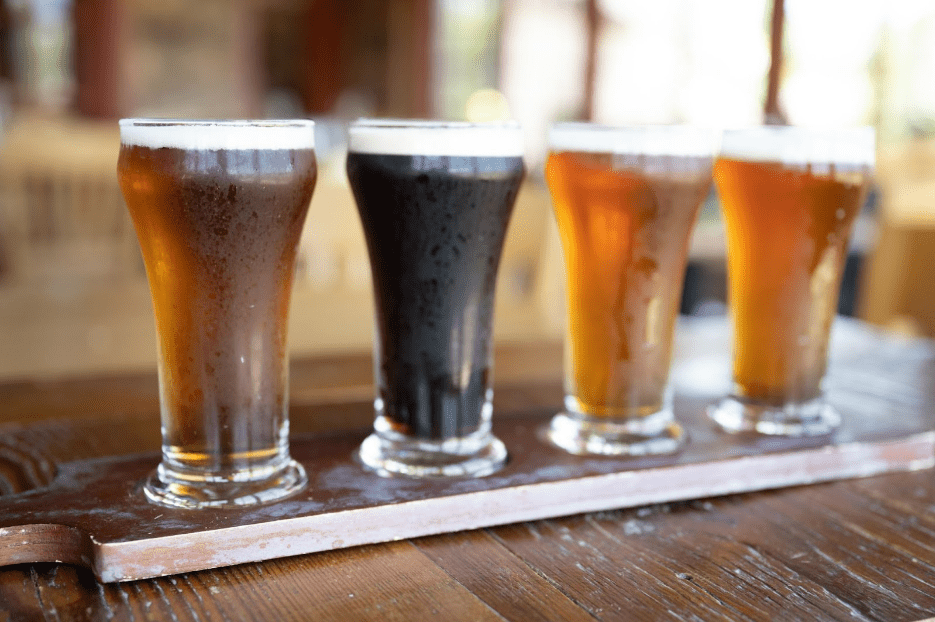The image is a color photograph in landscape orientation, capturing a flight of four beer schooners arranged side by side on a narrow wooden plank with a handle on the bottom left corner, serving as a tray. Each glass is tall, clear, and fluted toward the top, showcasing varied types of brew. From left to right, the first beer is a cloudy dark ale, followed by an almost black stout or dark brown ale, and two amber-colored beers which may include a Pilsner. All beers have a generous white foam head indicative of freshness. The plank and the glasses rest on a dark, rustic wooden table, and the ambient setting in the background, slightly out of focus, appears to be a lively restaurant or bar with windows in the top right. The photograph is a detailed, representational depiction of a beer tasting flight.